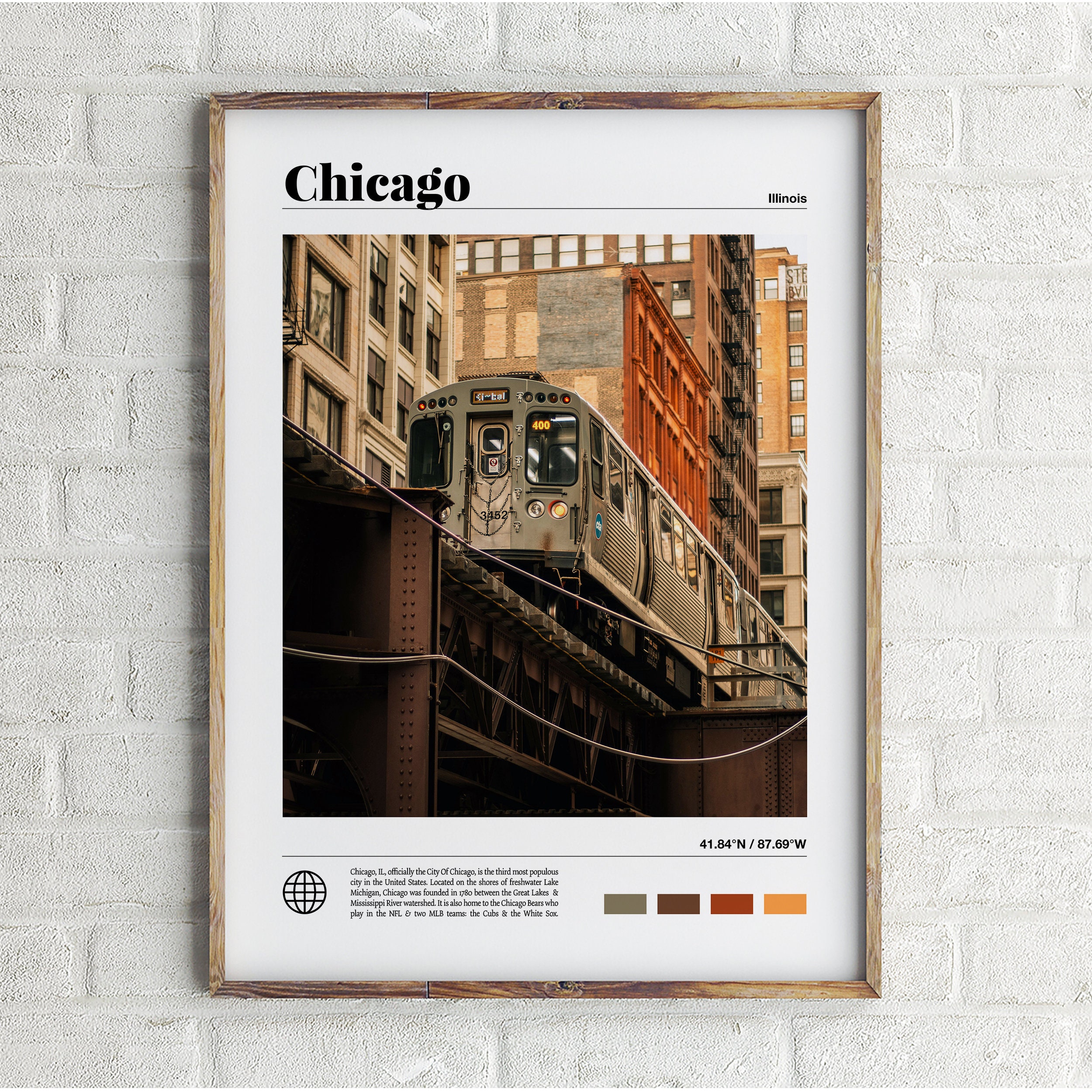The image features a whitewashed brick wall adorned with a framed picture. The frame is slender and wooden, encapsulating a visually engaging art piece. Central to the image is the word "Chicago" prominently displayed in bold black letters, accompanied by the smaller text "Illinois" in a matching black font. 

The focal point of the picture is a vivid, colored representation of a quintessential train navigating through downtown Chicago. The train bears the number "400" and is further identified by "3452." The backdrop consists of brick buildings, likely office complexes or apartment dwellings, viewed from a low angle as the train traverses an industrial-style bridge overhead.

At the bottom of the picture, geographic coordinates are listed, accompanied by an icon of a globe. Text beneath details key facts about Chicago, describing it as the third most populous city in the United States, located along the shores of Lake Michigan. The passage notes the history of Chicago, founded circa 1780, situated between the Great Lakes and the Mississippi River watershed, and mentions that the city is home to the NFL’s Chicago Bears and MLB’s Cubs and White Sox.

Flanking the main image are four rectangles in diverse hues: a grainy gray, brown, red, and a yellowy-orange. These color swatches mirror the colors found in the buildings depicted within the photograph, adding an additional layer of context to the visual narrative.